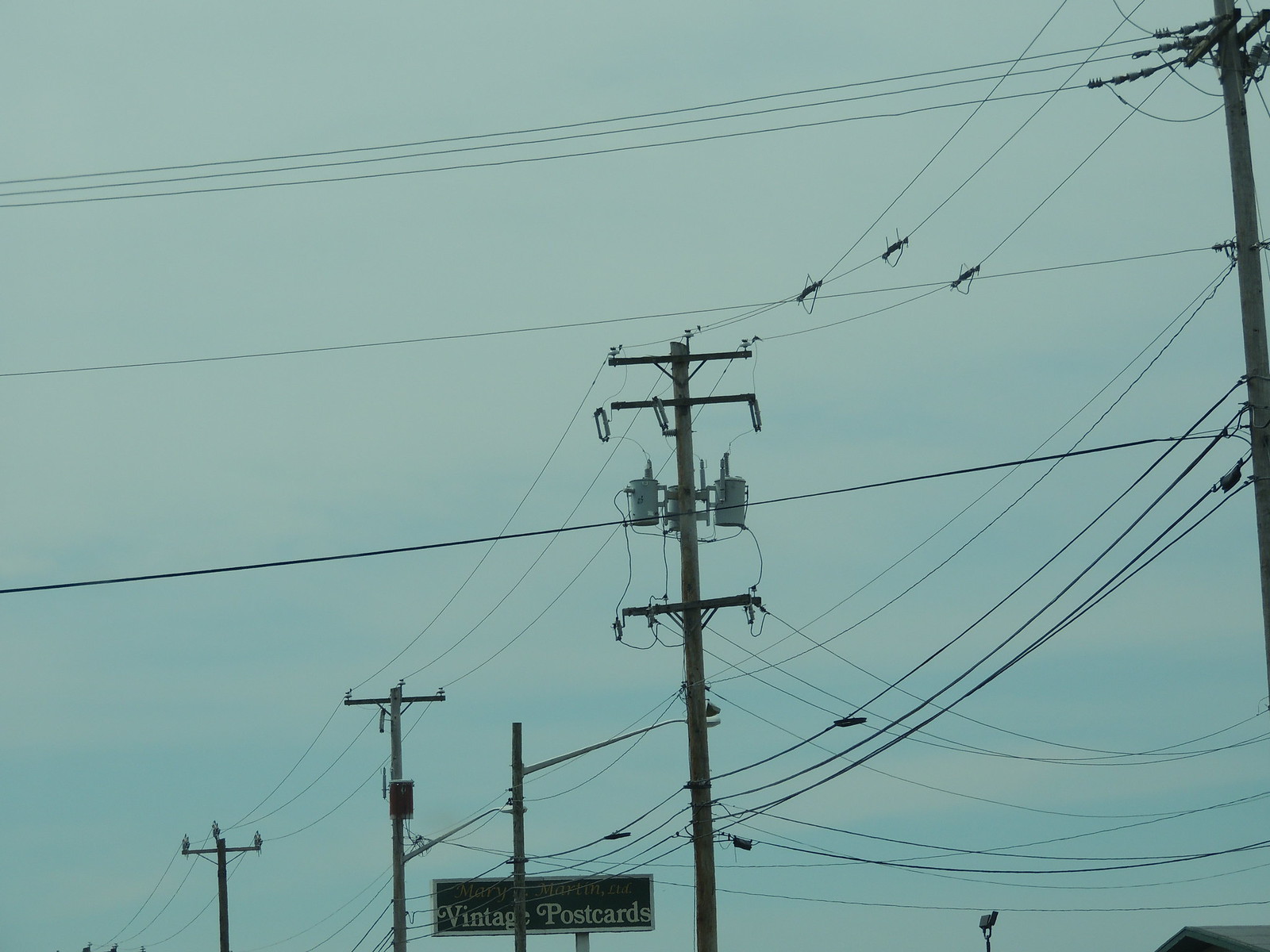This photograph, taken outdoors, captures a network of power lines against a predominantly blue sky with light, wispy clouds, giving a slightly overcast appearance. Four towering poles are lined up across the frame, creating a web of interconnected lines. These lines, silhouetted in black, stretch horizontally and dip between poles, creating an intricate pattern. Midway down the image, a retro sign reading "Mary Martin LTD Vintage Postcards" is nestled among the wires, its white script standing out against the backdrop. Just visible on the right edge of the frame is the sliver of a building's roof, adding a touch of urban context to the scene.